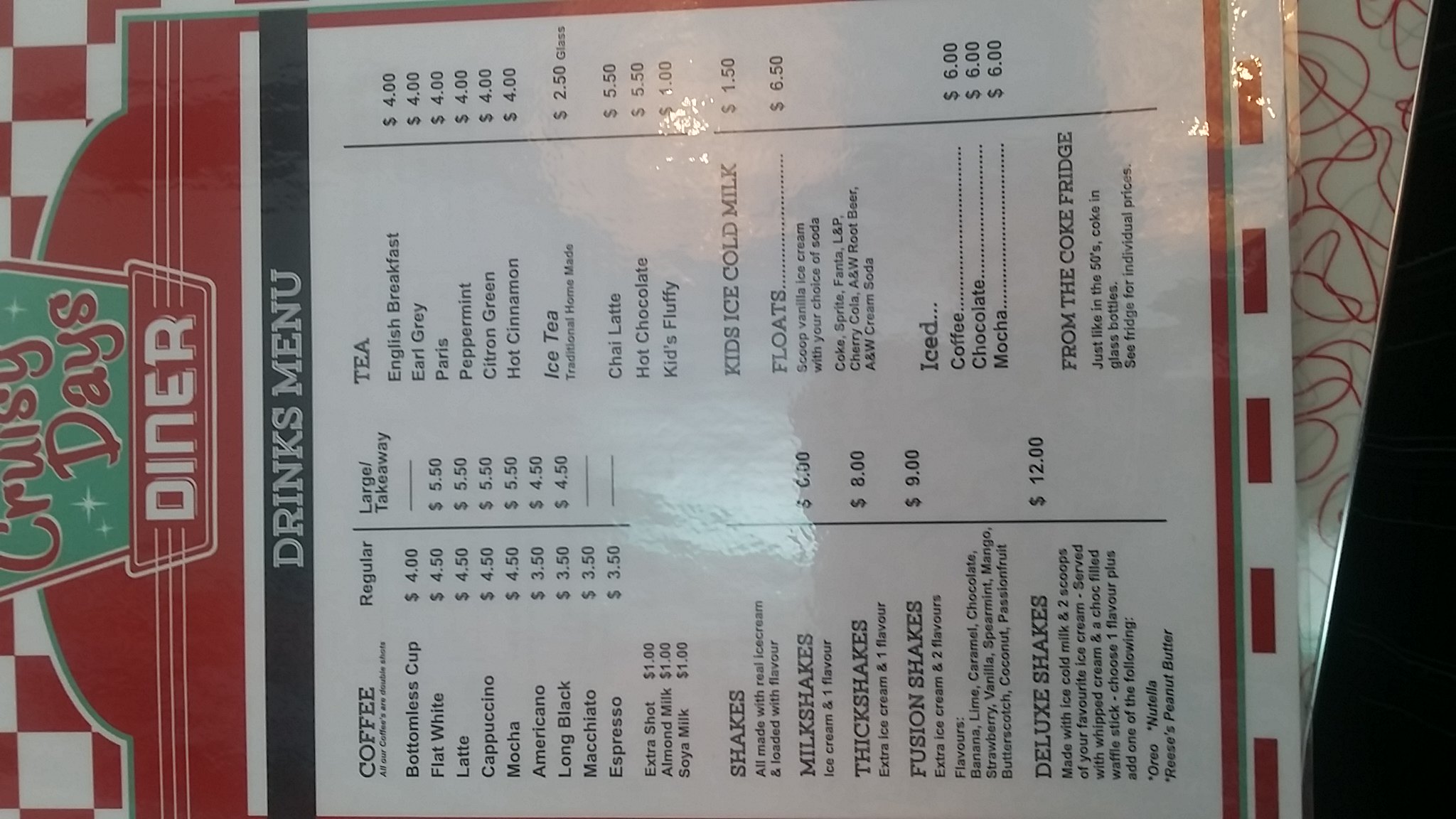The image features a menu that is positioned on a table and angled to the left by 90 degrees. The top section of the menu is slightly cut off, but it appears to read "Cruisey Days" or "Cruisy Days" and "Day's Diner." The menu highlights various drink options, such as coffee, tea, shakes, milkshakes, thick shakes, fusion shakes, and deluxe shakes. 

Under the tea category, the menu lists iced tea, chai tea, kids' cold milk, floats, iced coffee, chocolate, and mocha. Additionally, there is a mention of items available from the "cookie fridge," described as being reminiscent of the 1950s with options like a cookie and a glass. The menu also notes a "bottle sea fridge" for individual prices. The menu itself is predominantly white with red and light green squiggly lines adorning it.